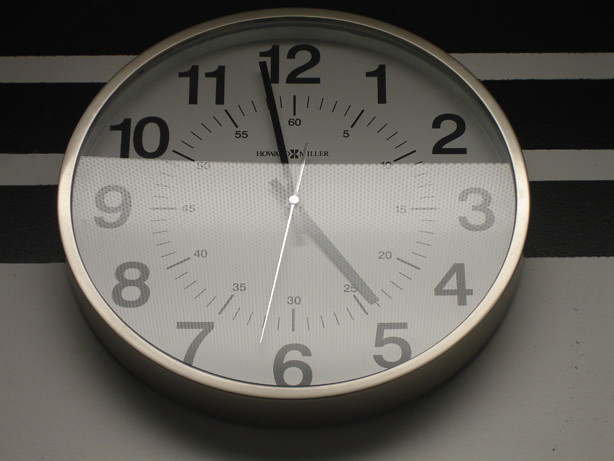This photograph captures a wall clock taken from a low angle, as if the viewer is standing on the floor looking up. The clock is mounted on a wall adorned with thick diagonal stripes: alternating bands of black and gray. The lower portion of the wall is entirely gray, leading up into the striped pattern. The clock is circular with a metallic, silver frame that protrudes slightly from the wall. The face of the clock is a stark white, encased in glass, with bold black numerals marking the hours. The hour hand and minute hand are black, positioning the time at approximately 4:58, while the second hand is a silvery metallic color. Within the clock face, a smaller ring with black dashes and numbers marks the seconds. The clock, manufactured by Howard Miller, casts a drop shadow beneath it while reflecting light on its lower half, creating a visually dynamic interplay of light and shadow.